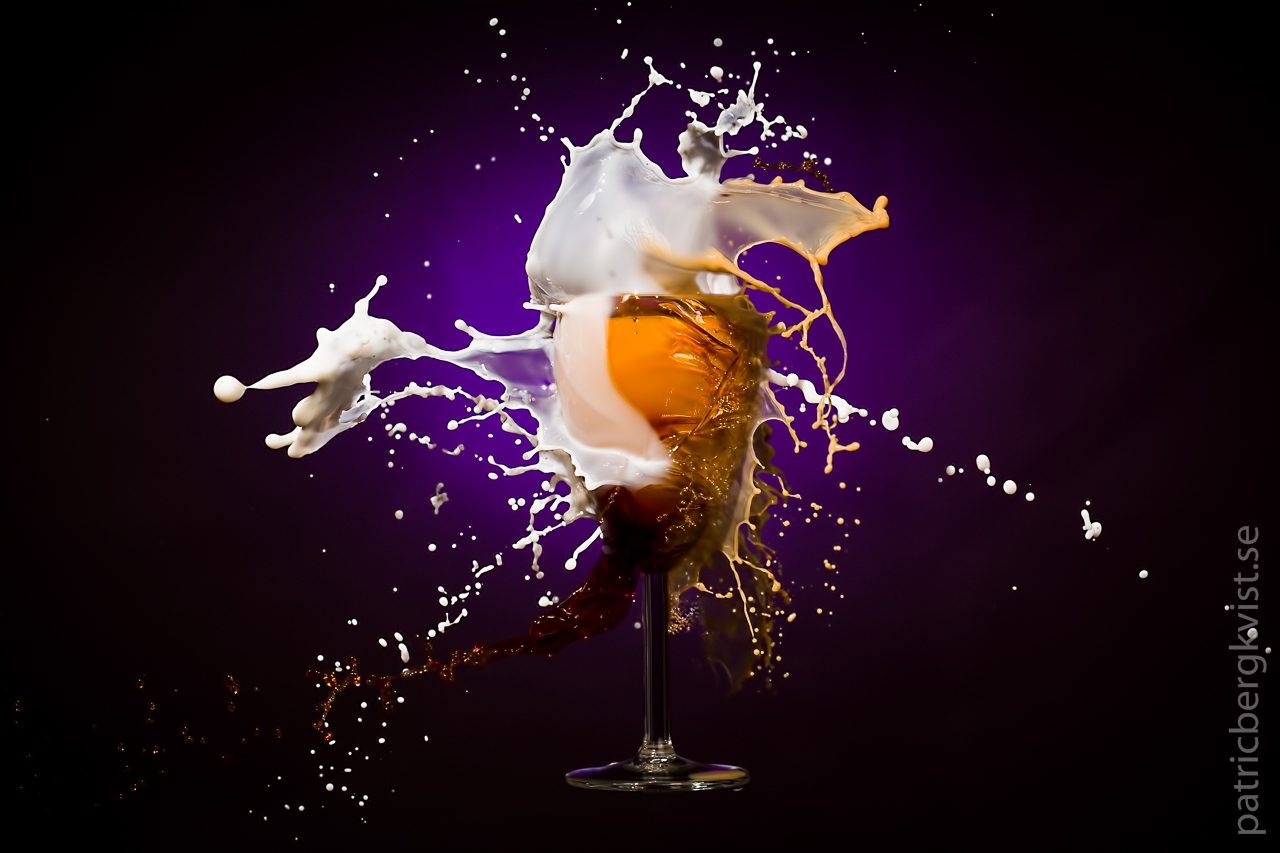The image features a stylized depiction of a goblet-shaped wine glass with a stem, set against a dark black background that gradates into a purple circle in the middle. The glass, which has a golden or amber hue, appears to be cracked and shattered at the front but still maintains its shape. From the glass, a white, milk-like liquid bursts forth in a dramatic explosion, splashing wildly in all directions with droplets resembling splatter paint. The scene captures an intense moment of action, with small grains of gold scattered in the background, adding to the visual spectacle. The bottom right corner of the image bears the text "patricebergviste.se", adding a hint of a professional photoshoot context.